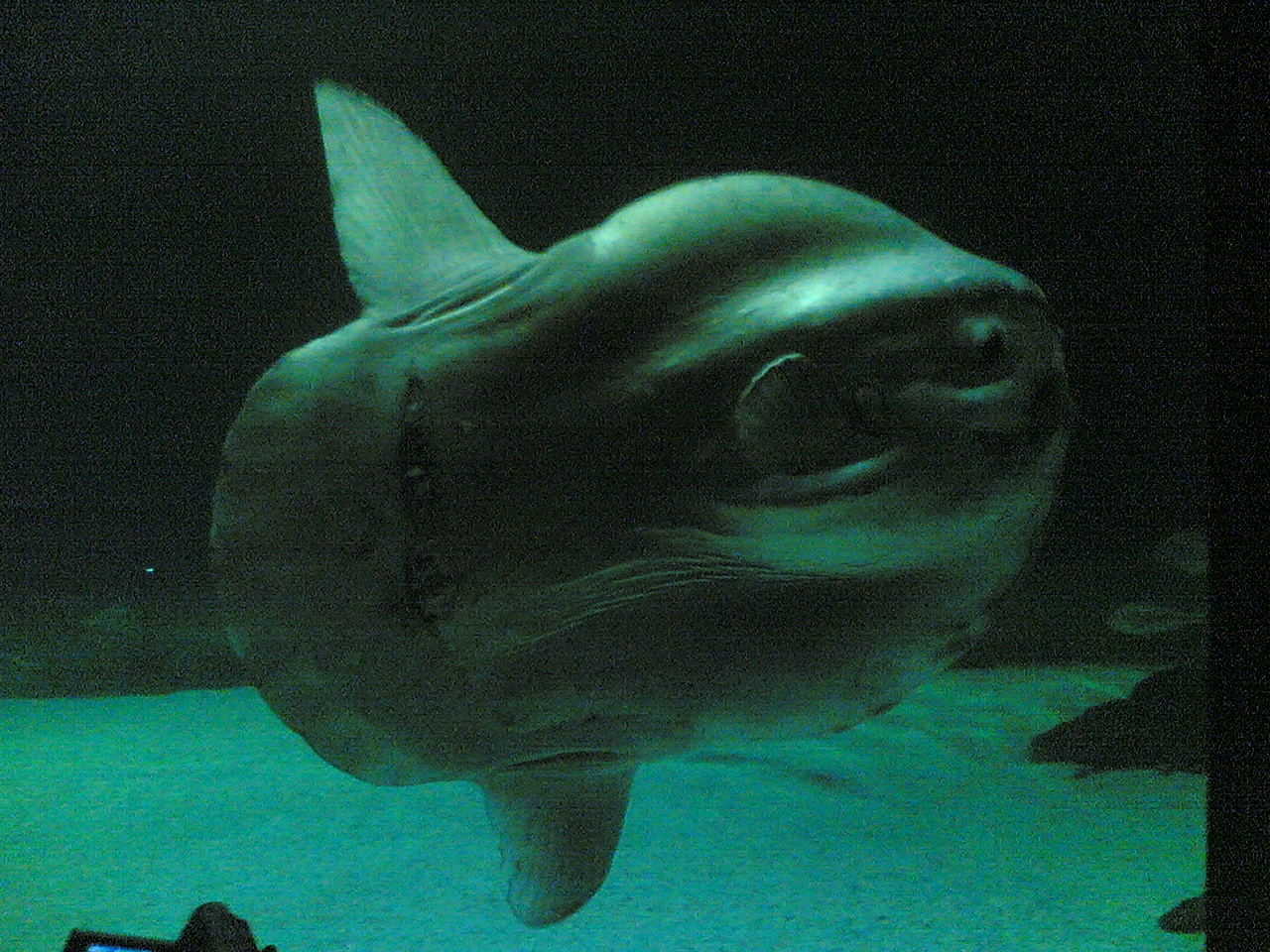The image is an underwater photograph, presented in landscape orientation, depicting a large, unidentified fish approaching the surface of a glass tank. The fish, which might be a dogfish or ocean sunfish, is oriented towards the right and features a dorsal fin on top, a ventral fin below, and smaller fins near its front. It has a distinctive rounded body and bulging eyes, giving it a somewhat blob-like appearance. The photograph, likely taken in a low-light aquarium setting, has a grainy and slightly blurry quality, with the illuminated tank exhibiting a greenish-blue hue. The sandy bottom of the tank is visible, dotted with a few rocks and small fish in the bottom right corner. The background behind the fish is a dark, almost black expanse, heightening the murky, mysterious atmosphere of the scene.